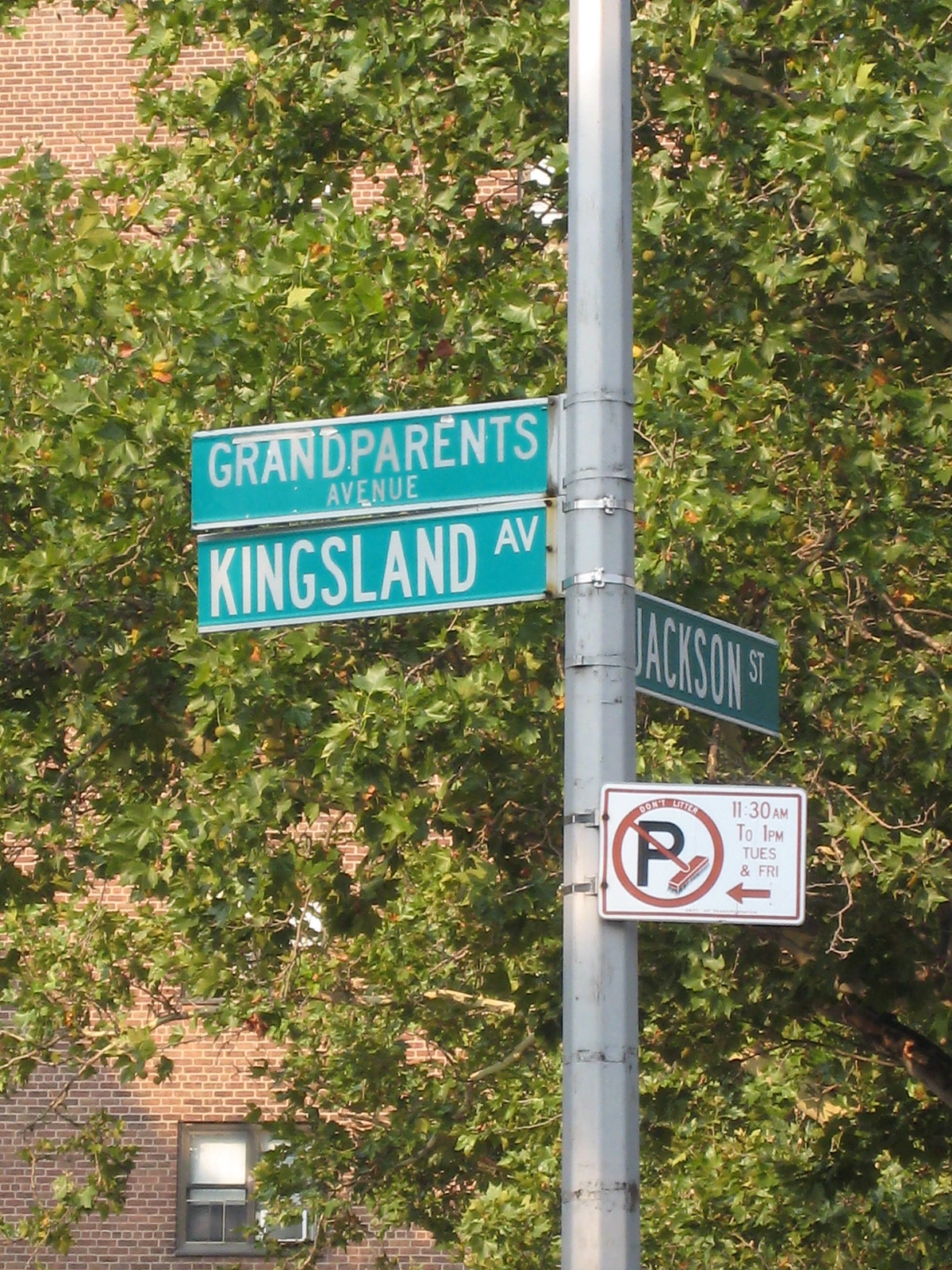On this street corner, a brick building with a couple of visible windows stands prominently. Adjacent to it, a large green tree provides ample foliage. A sturdy silver metal pole is affixed to the ground, featuring a white sign with a red circle and a black "P" crossed out by a red line, indicating no parking in this area, accompanied by specific time restrictions. Additionally, three green street signs project from the pole: one pointing towards Grandparents Avenue, another towards Kingsland Avenue, and the last one in the opposite direction indicating Jackson Street.